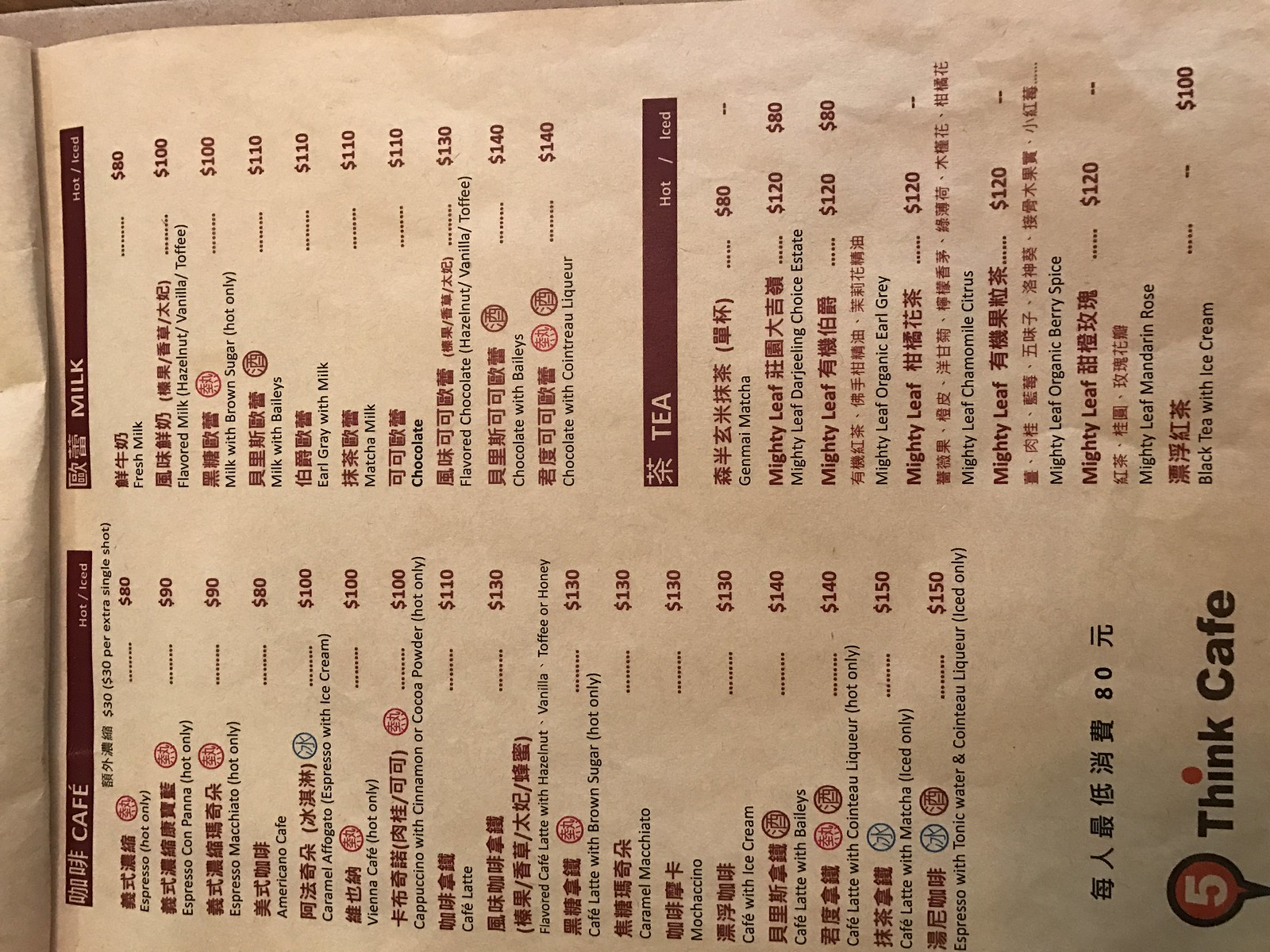The image displays a cafe restaurant menu, oriented sideways. The menu predominantly features red text that lists the names of various items, primarily written in Chinese, possibly Japanese. Certain sections of the menu are organized under red headers with white text, some of which are in English, such as "Milk" and "Tea." The items are described in black text, which appears to be in English, and the prices are indicated in US dollars. At the bottom of the menu, a distinctive black bubble with a white number "5" is pointed downward. Adjacent to this, the name "Think Cafe" is displayed in black text, with the "i" stylized as a red dot. The background of the menu is a vibrant red, providing a striking contrast to the text.